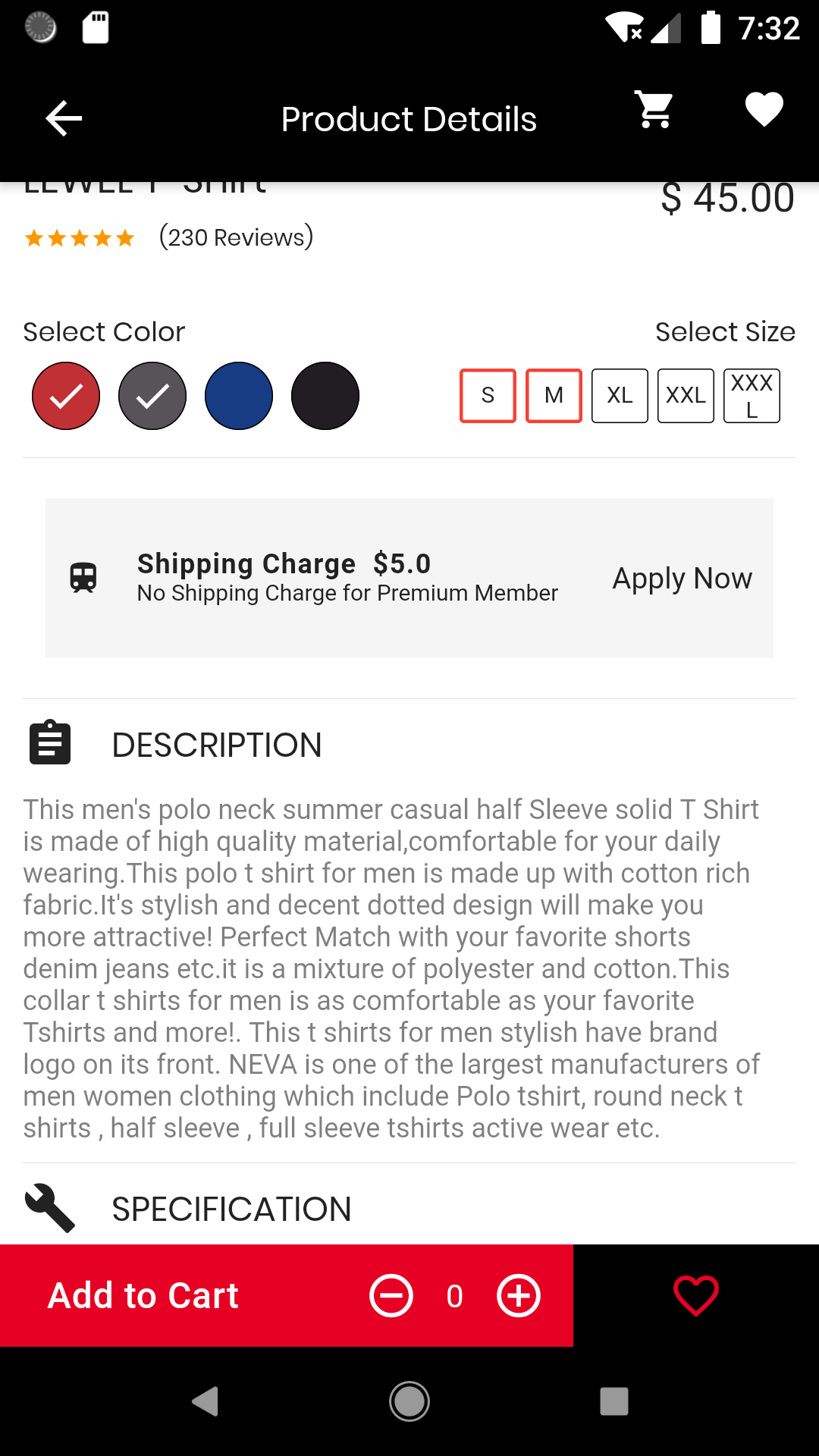This image is a screenshot of a cell phone displaying a product details page for an item. The timestamp on the photo indicates it was taken at 7:32. At the top, there is a black header with "Product Details" written in white font. To the right of this heading are icons for a shopping cart and a heart, symbolizing favorites.

Beneath the header, the background changes to a white canvas. The product image occupies about 80% of the space but is partially obscured, making the product name unreadable. The visible price of the item is $45. The product has received 230 reviews and is available in four different colors. The available sizes are Small (S), Medium (M), Extra Large (XL), XXL, and XXXL. The sizes Small and Medium are highlighted in red, indicating their selection.

Further down, the page displays a shipping charge of $5, with an option for free shipping for premium members, who are prompted to "Apply Now."

The product description reads:
"This men's polo neck summer casual half-sleeve solid t-shirt is made of high-quality material, comfortable for daily wear. This polo t-shirt for men is made with cotton-rich fabric. Its stylish and decent dotted design will make you more attractive. Perfectly matches with your favorite shorts, denim, jeans, etc. It is a mixture of polyester and cotton. This collar t-shirt for men is as comfortable as your favorite t-shirts and more. This t-shirt style features a brand logo on its front. NEVA is one of the largest manufacturers of men's and women's clothing, including polo t-shirts, round neck t-shirts, half sleeve, full sleeve t-shirts, active wear, etc."

Below the description, there is an icon with the word "Specifications," followed by the "Add to Cart" option, which currently shows a quantity of zero.